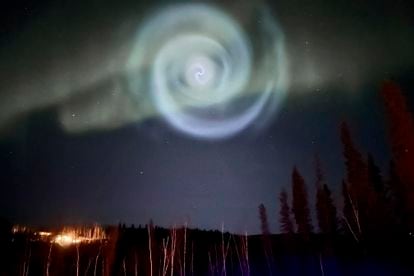In this captivating night scene, a dramatic purple and teal spiral dominates the dark blue sky, its mesmerizing pattern swirling gracefully from the center towards the left, then looping back up and down with subtle variations. Yellow streaks punctuate the spiral near the upper left, adding a touch of luminosity to the atmospheric tableau. The background is an almost pitch-black sky, creating a stark contrast to the vivid colors. Below the celestial display, the edge of the Earth is visible, grounding the ethereal vision. On the right side, faint silhouettes of plants reach upwards, while the bottom left is illuminated by a large bonfire, its bright orange flames casting a warm glow and creating lines that extend horizontally. This photo beautifully captures a scene reminiscent of the northern lights, blending natural wonder with an almost surreal quality.